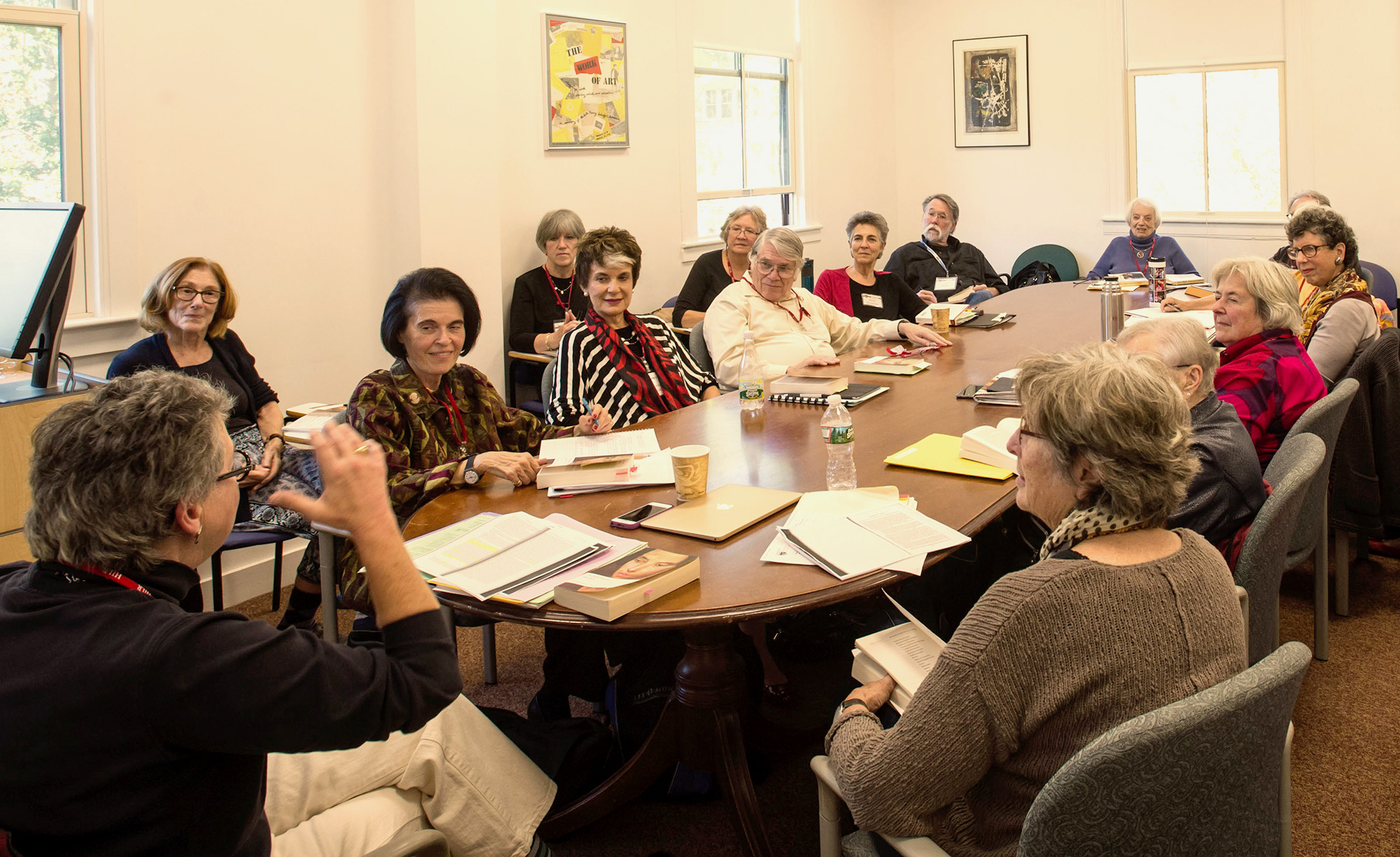This photograph depicts a small, indoor conference room filled with over a dozen middle-aged to elderly individuals, mostly women, gathered around a long, brown wooden table. The focal point is an elderly man with short gray hair and small round glasses, wearing a black long-sleeved shirt and white trousers. He stands at the bottom left corner of the image, facing the group with his back to the camera, noticeably engaged in conversation. The table is adorned with several open papers, paperback novels, and a water bottle, indicating a possible book discussion or a meeting. The participants, seated in gray fabric-lined chairs, also appear to have name tags or lanyards. The room features white walls with multiple windows—a pair on the left and one on the right—letting in natural light. In the background, a few more individuals can be seen sitting on chairs away from the main table, adding to the collaborative atmosphere of the setting. A computer system is placed beside one of the windows on the left side of the image.